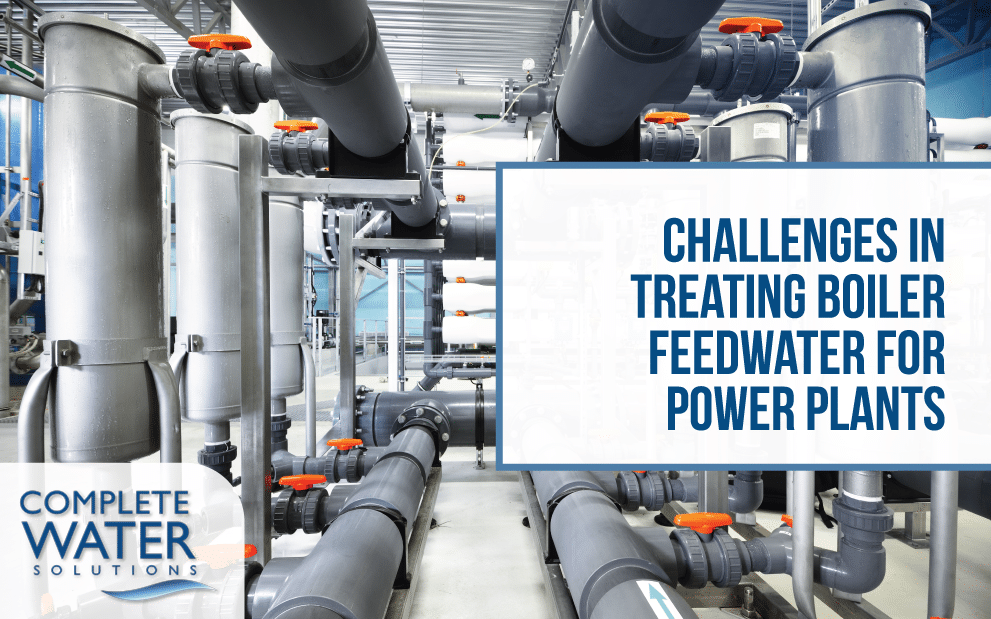The image portrays a clean and modern industrial setting, likely inside a power plant, featuring an array of large gray pipes, ducts, and canisters connected by various orange-handled valves. Dominated by a sterile and structured look, the facility houses intricate piping systems connected to sizable drums. Two white rectangles with blue text overlay the image: the one in the lower left, slightly see-through and rounded at the upper right corner, displays the text "Complete Water Solutions" beside a blue swirl with a white underside. The rectangle on the right, bordered in blue with right-aligned text, reads "Challenges in Treating Boiler Feed Water for Power Plants." The background's walls or possible window panels are blue, adding to the industrial ambiance.